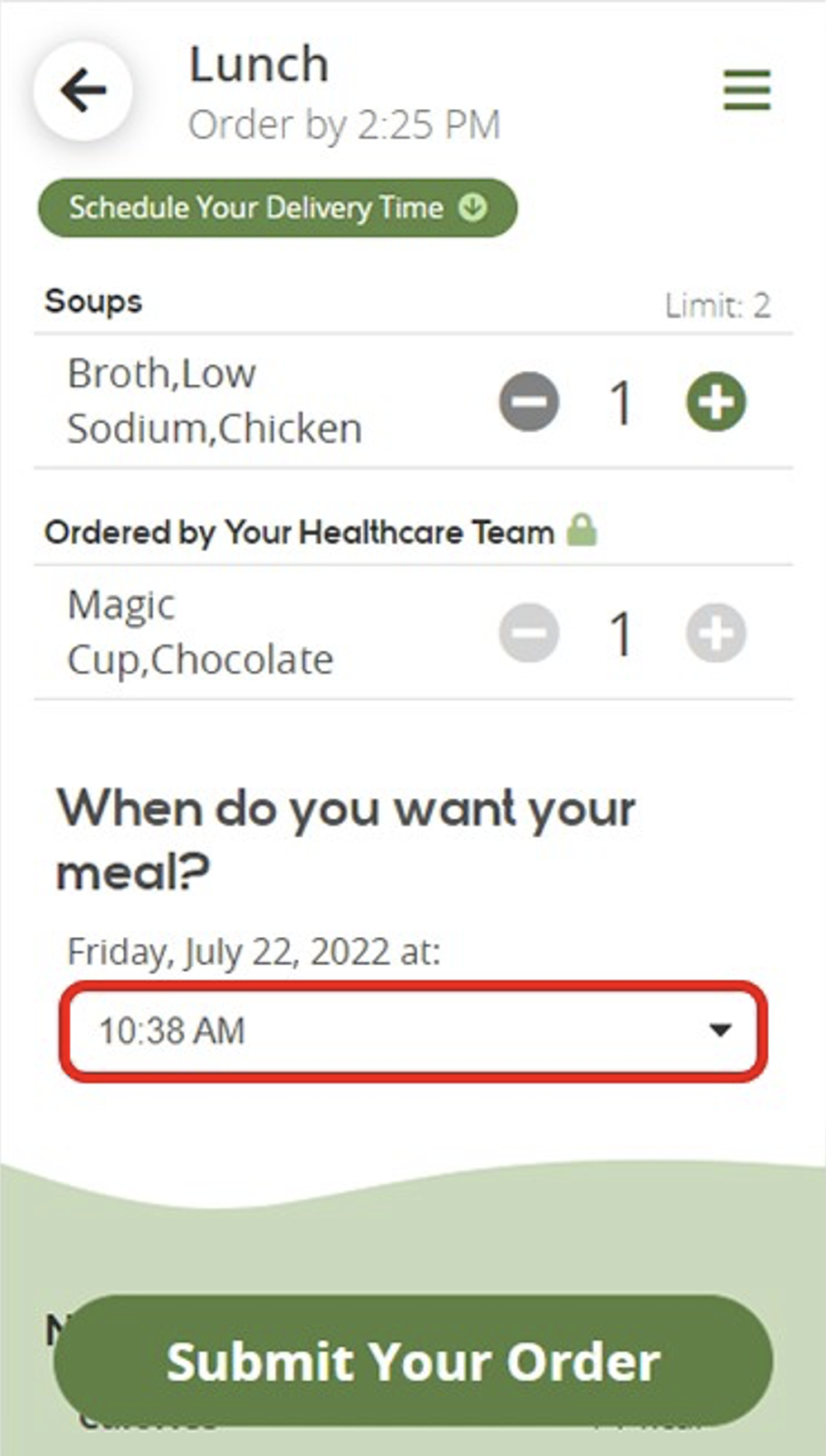**Detailed Caption for the Screenshot from a Food Ordering App**

The image displays a smartphone screen showing a user interface of a food ordering app with a white background and green accents. At the top, the order is categorized as a "Lunch Order" in bold text. Below this header, in grayed-out text, it indicates that the order must be placed by "2:25 p.m." 

A green header button with a drop-down arrow is visible just below this, labeled "Schedule Your Delivery Time." This button likely opens further options for scheduling the delivery.

The lunch order section lists two items. The first item falls under the "Soups" category, marked with a "limit 2" restriction at the far end. Within this section, "Broth, Low-Sodium Chicken" is listed, showing that one unit has been ordered. There are plus and minus icons present beside the quantity, enabling the user to adjust the number of soups ordered.

Under a separate section labeled "Ordered by Your Healthcare Team," the item "Magic Cup, Chocolate" is listed, with one unit ordered. This item has no quantity adjustment features displayed.

Another section beneath these items asks, "When do you want your meal?" followed by a specified date, "Friday, July 22nd, 2022." A time selector is provided, showing the chosen delivery time as "10:38 a.m.," highlighted and circled in red to indicate the selected delivery time.

At the bottom of the screen, a light green section features a large, wide green button with white text that reads "Submit Your Order," allowing the user to finalize their meal order.